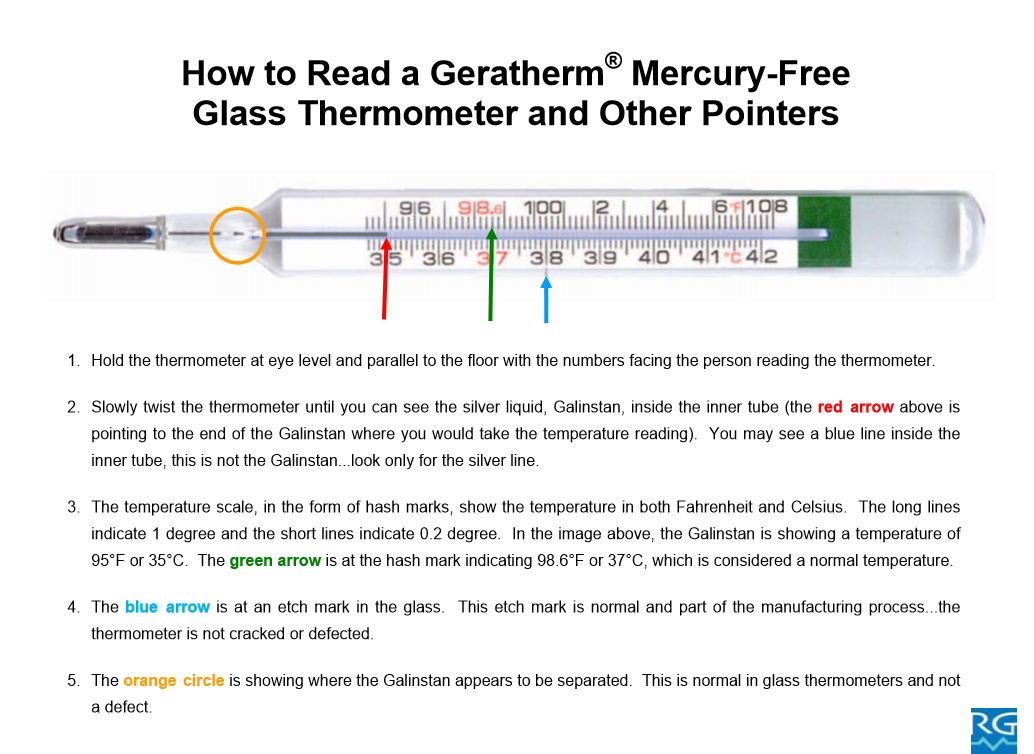The image is a detailed diagram on how to read a Gerotherm mercury-free glass thermometer. At the top, it says "How to Read a Gerotherm Mercury-Free Glass Thermometer and Other Pointers," with a registered trademark symbol next to “Gerotherm”. 

The photograph of the thermometer shows a thin glass tube that spreads out slightly as it extends. A key feature inside the thermometer is the silver liquid, which is Galistan, used instead of mercury. The thermometer displays temperature scales in both Fahrenheit at the top and Celsius at the bottom. Long hash marks indicate one degree increments, while short hash marks indicate 0.2 degree increments.

Five key instructions and several colored indicators guide the reader:

1. **Hold the Thermometer Properly**: Hold the thermometer at eye level and parallel to the floor with the numbers facing you.
2. **Twisting to See the Galistan**: Twist the thermometer slowly until you can see the silver liquid (Galistan) inside the inner tube. There may be a blue line inside the tube, but this is not the Galistan. Look only for the silver line. 
3. **Reading the Temperature**: The temperature scale uses hash marks to show both Fahrenheit and Celsius. In this image, the Galistan shows a reading of 95°F (35°C). The red arrow points to the end of the Galistan line used for the temperature reading.
4. **Identifying Normal and Defect-Free Features**: The green arrow indicates the hash mark showing 98.6°F (37°C), which is considered a normal temperature. The blue arrow points to an etch mark in the glass, which is a standard part of the manufacturing process and not a defect.
5. **Separations in Galistan**: The orange circle highlights where the Galistan appears separated, which is normal for glass thermometers and does not indicate a defect.

The bottom of the image contains a square logo with the letters "RG" in white over a blue background.